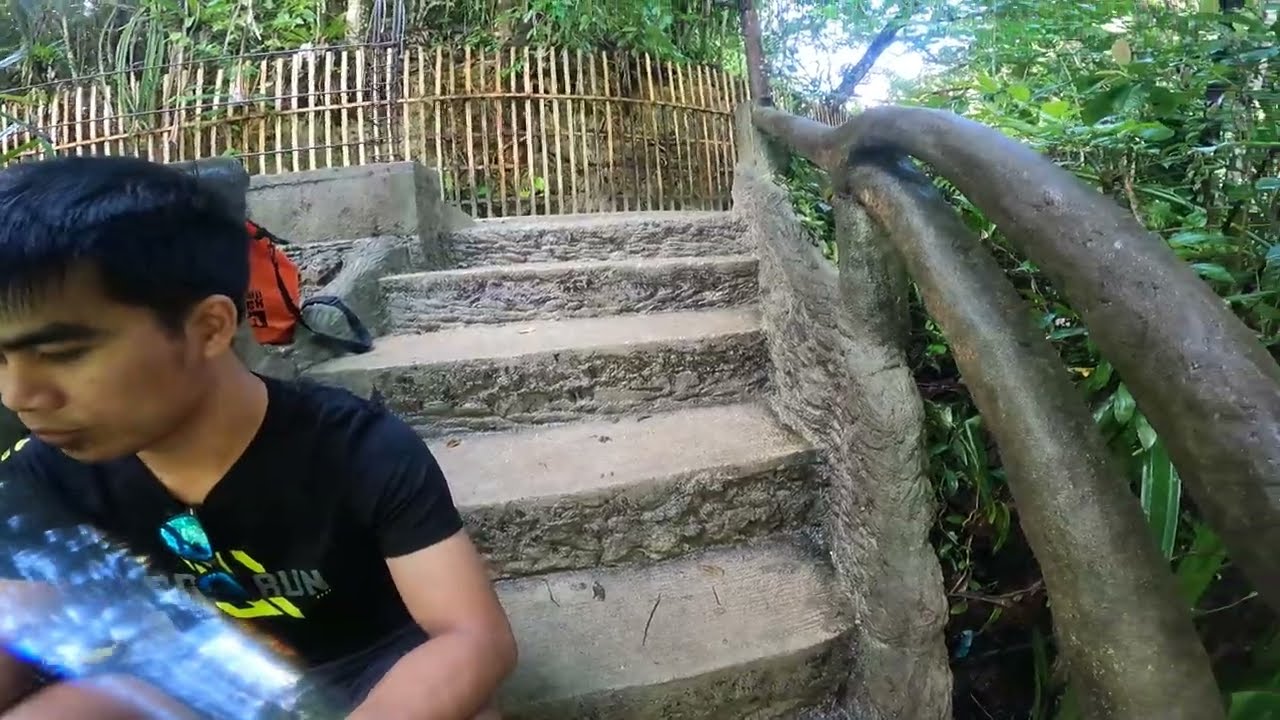The photograph captures a man with short black hair and dark eyebrows sitting on aged, rough cement steps that lead upward to the right. He sports a black t-shirt with partially readable white lettering and a possible yellow pattern that is obscured by lens flare, along with sunglasses hanging from his collar. The man, who has tan skin, holds a blurry item, likely a water bottle. Behind him is a red backpack with a black handle. The steps, which appear old and worn, are accompanied by a cement handrail on the right melding into a backdrop of abundant greenery. The surroundings feature a wooden fence made from thin slats rising from the top of the steps. A patch of trees and lush foliage behind the fence and handrail allows specks of light and sky to filter through. The image has a slight fisheye or GoPro lens effect, adding a warped appearance to the scene.